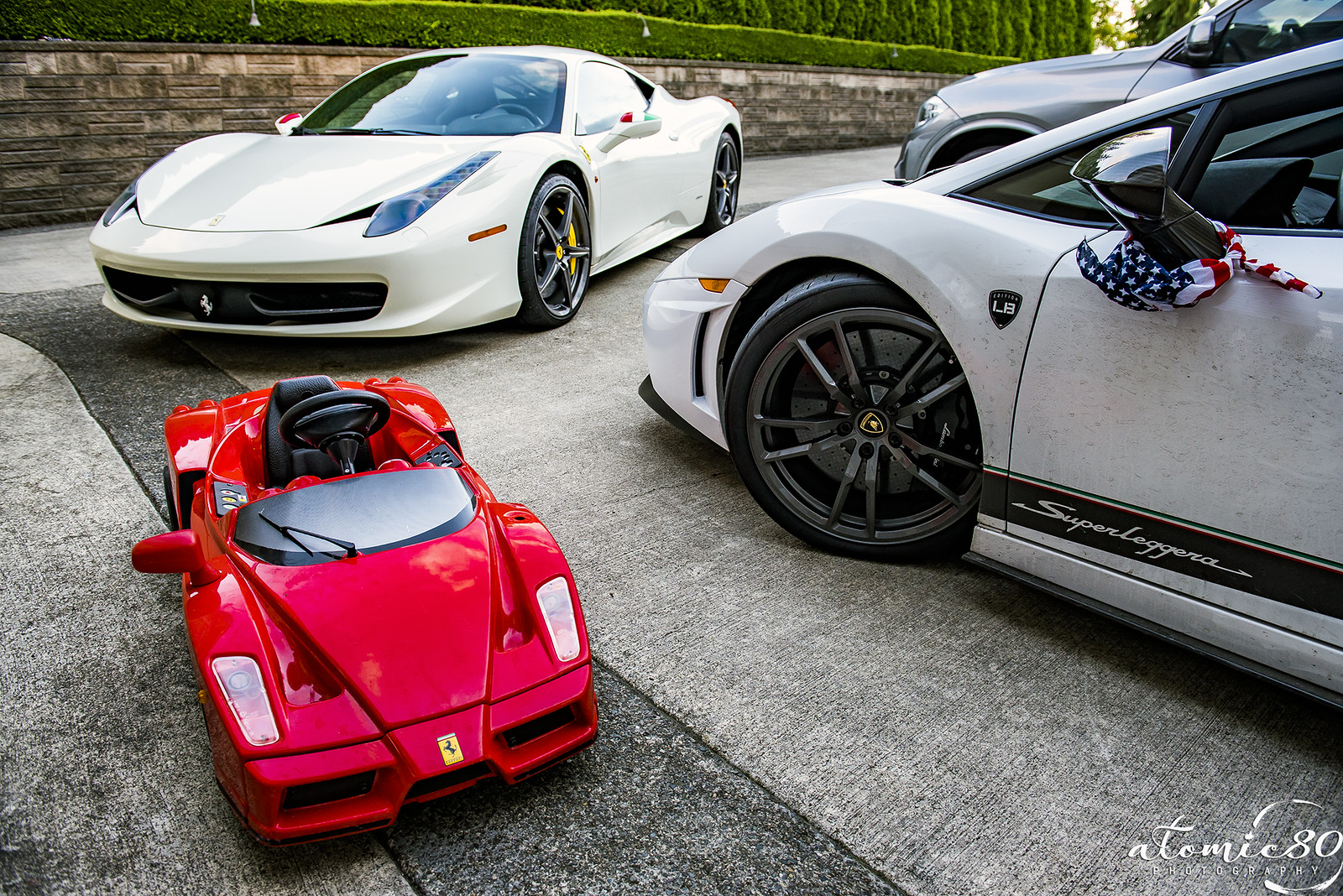This photograph captures a diverse collection of vehicles parked on a light gray, cement-like area that almost resembles carpeting. Prominent in the image are two luxury cars set against a backdrop featuring a wooden fence, a green hedge, and some trees. The first car on the right is a Lamborghini Superleggera, noted for its white body adorned with speckles of dirt or mud, low-slung frame, and an American flag bandana wrapped around its distinctly black chrome side-view mirror. The Lamborghini's front end, positioned from the right, dominates the scene. Directly behind it is another opulent white car, identified as a Ferrari, akin to a street-legal race car. Both vehicles exhibit high-end design features and emphasize the luxury theme of the setting. Additionally, to the lower right-hand corner lies a detailed, child-sized red Ferrari replica with the iconic Ferrari logo on its hood. Despite its smaller scale, it is a meticulous mimicry complete with lights, windshield wipers, and an open convertible structure. Behind this toy vehicle stands a large gray SUV, blending into the setting while enhancing the variety of the cars presented. The scene's composition and background elements create a layered, vibrant snapshot of various automobiles ranging from high-end supercars to playful replicas.